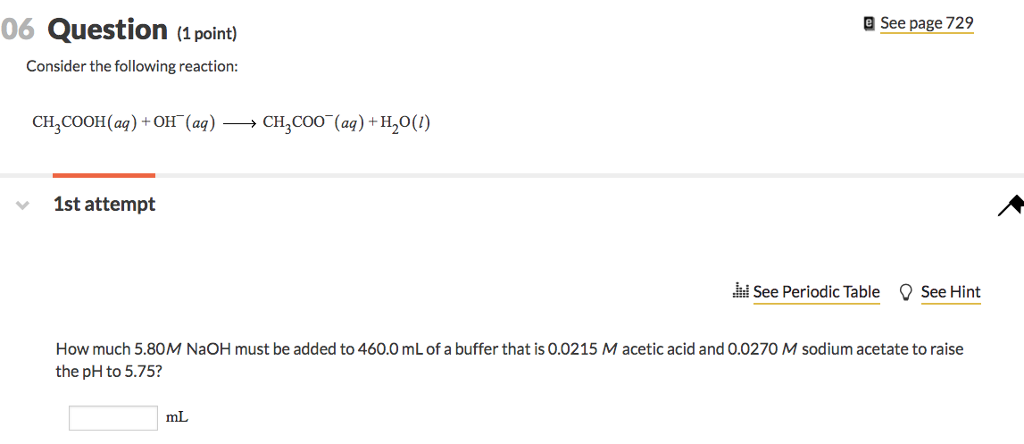**Detailed Caption:**

This is a detailed screenshot in landscape mode featuring a predominantly white background with a structured layout in two main sections. 

**Upper Section:**
- **Top-Left Corner:** In this area, there is a label in gray text that reads "06," followed by a bold black text "QUESTION," and then "(1 point)" in parentheses.
- **Top-Right Corner:** There is an "E" enclosed within a square, next to an underlined hyperlink in orange text that reads "See page 729."
- **Main Content:** Below the "QUESTION" label, there's a sentence in black text that says "Consider the following reaction:"
- **Chemical Equation:** The reaction is displayed as "CH₃COOH (aq) + OH⁻ (aq) → CH₃COO⁻ (aq) + H₂O (l)."

A thin gray line separates the upper section from the bottom section.

**Bottom Section:**
- **Left Side:** The phrase "First Attempt" is in bold text, above which there's an orange line and a drop-down arrow.
- **Right Side:** The options "See periodic table" and "See hint" are interactive links, with an additional option to flag the question.
- **Question:** The prompt following these options asks, "How much 5.80 M NaOH must be added," followed by the continuation of a detailed numerical question.